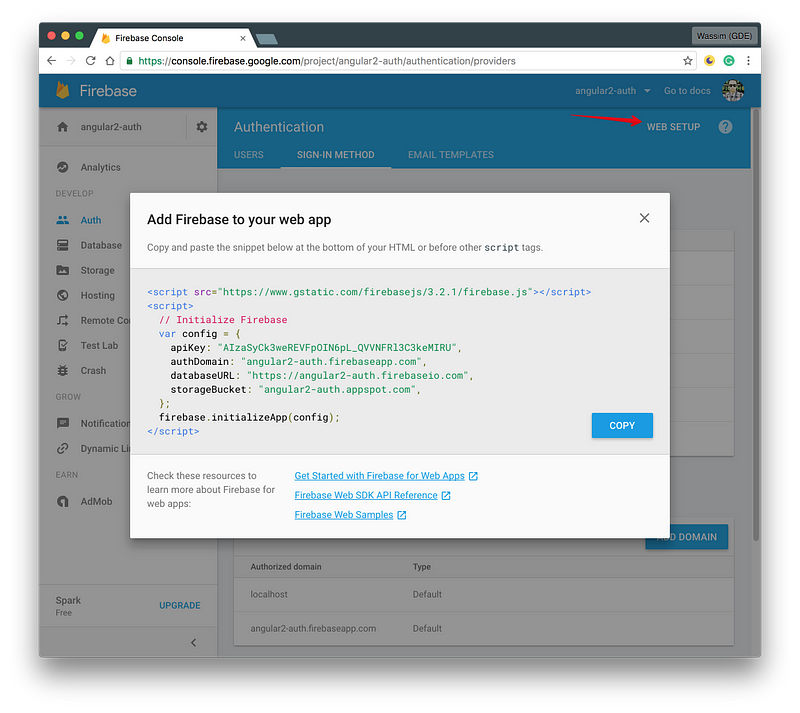The on-screen image is a screenshot of the Firebase Console on a web browser. It features three colored control buttons at the very top: red, orange, and green, representing the standard close, minimize, and maximize buttons respectively. Just below these buttons is an open tab labeled "Firebase Console."

Directly beneath the tab label is a search bar containing the URL: consoles.firebase.google.com. Scrolling further down, the main content area displays a large, open white box situated in the center of the screen. In the top-left corner of this box, the text reads: "Add Firebase to your web app."

Below this header, there is an instructional line that states: "Copy and paste the snippet below at the bottom of your HTML or before other script tags." Under this instruction is a block of script text intended for backend configuration, comprised of various letters and symbols relevant to implementing Firebase.

At the very bottom of the white box, a section encourages users to explore further with the text: "Check these resources to learn more about Firebase for web apps." This is followed by three blue information bars, each providing a clickable link for additional information. The first bar reads: "Get started with Firebase for web app."